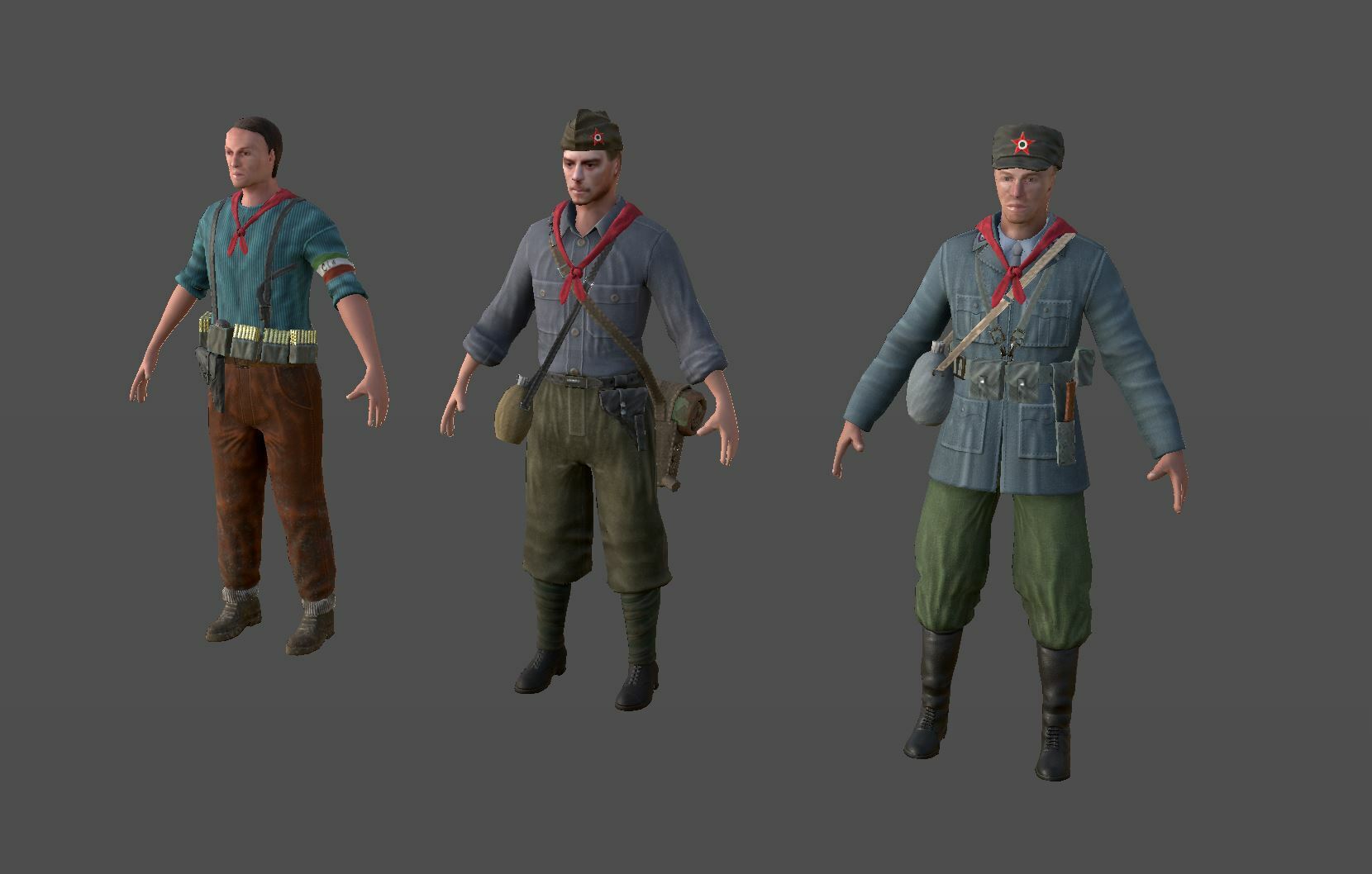This image is a 3D rendering showcasing three Caucasian male character models that appear to be soldiers or fighters, positioned against a gray-brown background. All three characters are depicted with their arms slightly away from their bodies, giving the appearance of a standardized pose typical of a character creation suite in video games or computer simulations.

Starting from the left, the first model is dressed in brown pants and boots, with a short-sleeved blue shirt that has trim detailing around the sleeves. He sports a red scarf tied around his neck and has a holster with an ammo belt around his waist. His short hair and caucasian features are clearly visible.

The middle character wears green boots, green pants which are tucked into the boots, and a gray shirt. He also has a red scarf tied around his head and a green military-style cap adorned with a red insignia over his left eye. This model is equipped with a canteen strapped across his chest, resting on his right hip, along with another small pack on his left hip, and he similarly has his arms out to his sides.

The third character on the right is outfitted in green pants, brown boots, and a blue jacket with multiple pockets. He also has a red scarf around his neck, a canteen over his shoulder, and a cap with a red star emblem. This character's jacket extends below his waist and he appears to have a belt across his midsection.

All three models share the commonality of wearing a red scarf, further emphasizing their possible association as soldiers or fighters. The rendering style and the somewhat plastic, unreal appearance of the characters suggest they are computer-generated images rather than photographs of physical dolls or figures.